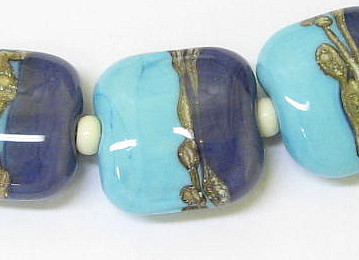This is a close-up photograph of a beaded piece, likely a necklace or bracelet, set against a pristine, flat white background. The image focuses on a sequence of three beads arranged in a line, with only the middle bead fully visible. Each bead is a rounded square shape, with a light blue bottom transitioning to a dark blue top, and adorned with an intricate gold design around its circumference. 

The central bead is vertically divided with a gold decorative design, featuring a top half of dark blue and a bottom half of light blue. This bead is smooth and shiny, suggesting a polished stone or glass material. The left bead is partially visible, showing a dark blue top and a hint of the gold design. Similarly, the bead on the right is also partially visible, primarily revealing its light blue bottom and a segment of the gold design.

Each of the main beads is connected by smaller white beads, which serve as connectors in the sequence. A shadow cast on the foreground indicates that the light source is coming from the upper left corner of the image, adding depth and enhancing the reflective qualities of the beads. The overall arrangement and detailing suggest an elegant and finely crafted piece, likely intended for wear as jewelry.